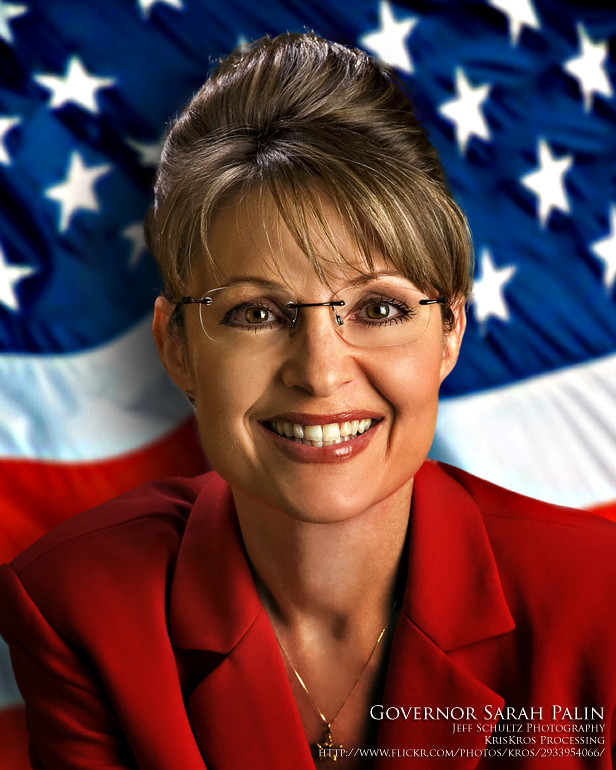This is a tall rectangular photograph of Sarah Palin, visible from the shoulders up against a backdrop of a close-up American flag. Palin, a governor, is a Caucasian woman with tan skin and short brown hair styled in a glossy updo with bangs swooping towards the bottom right. She wears rimless or subtly rimmed glasses, a shiny red suit jacket, and a thin gold necklace with a small gold pendant. Her bright red lipstick accentuates her broad smile, revealing both rows of her neat teeth. Behind her, the American flag appears wrinkled or wavy, with visible white stars on a blue field at the top, followed by a white stripe and beneath it, a red stripe. In the bottom right corner, in white all-capital letters, the text reads "Governor Sarah Palin," with a smaller block of text below that, which includes "Jeff Schultz photography" and "crisscross processing" along with a link.